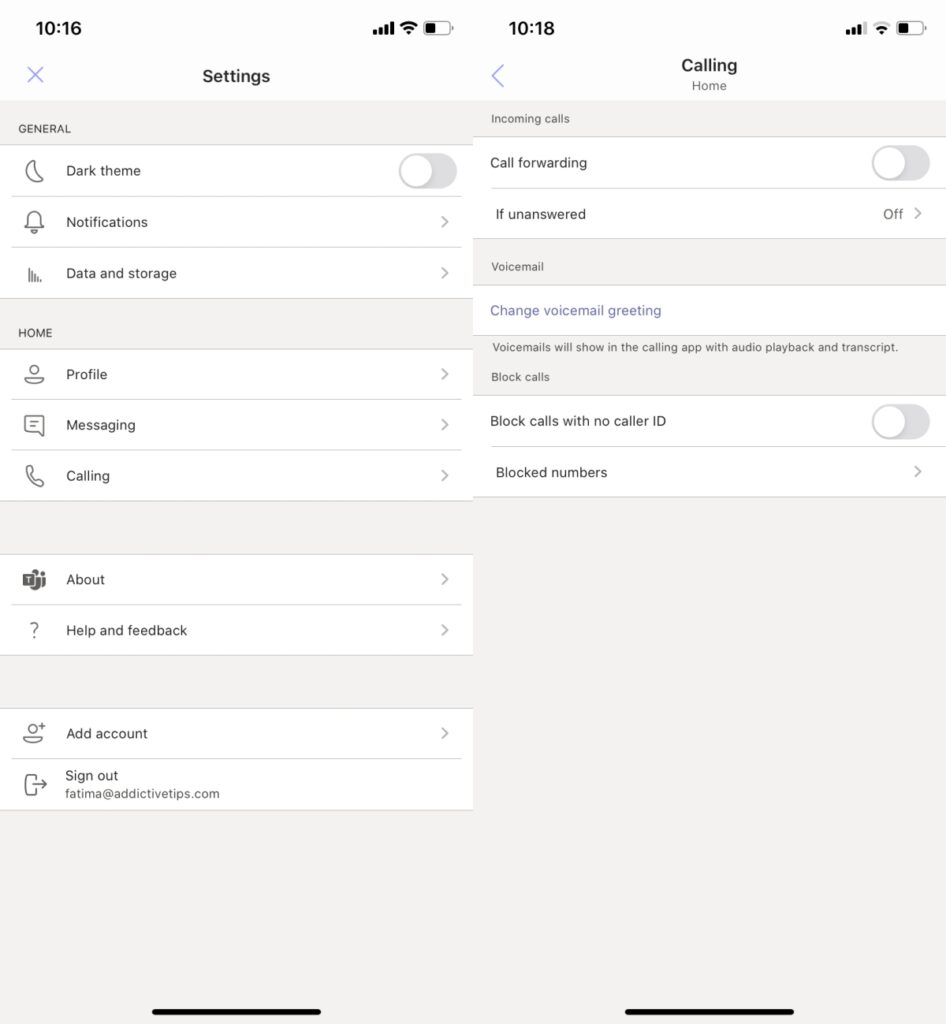This image showcases a composite of two screenshots side-by-side from a cell phone display. At first glance, the photos might appear as a single image, but a closer inspection reveals distinct details in both the left and right halves. The left screenshot was taken at 10:16 and depicts the phone's settings page. The settings include various options: "Dark theme" is toggled off, and below it, options for "Notifications," "Data and storage," "Home," "Profile," "Messaging," "Calling," "About," "Help," "Feedback," "Add account," and "Sign out" are listed sequentially.

On the right side, the screenshot, captured at 10:18, displays a page titled "Calling Home." This page contains options specific to call settings. "Call forwarding" is set to off, as is the "If unanswered" option. The "Voicemail" section suggests that users can "Change voicemail greeting," and mentions that "Voicemails will show in the calling app with audio playback and transcript." Towards the bottom, there is a section for managing blocked calls, labeled "Blocked calls with no caller ID," which is also turned off, alongside a list of "Blocked numbers."